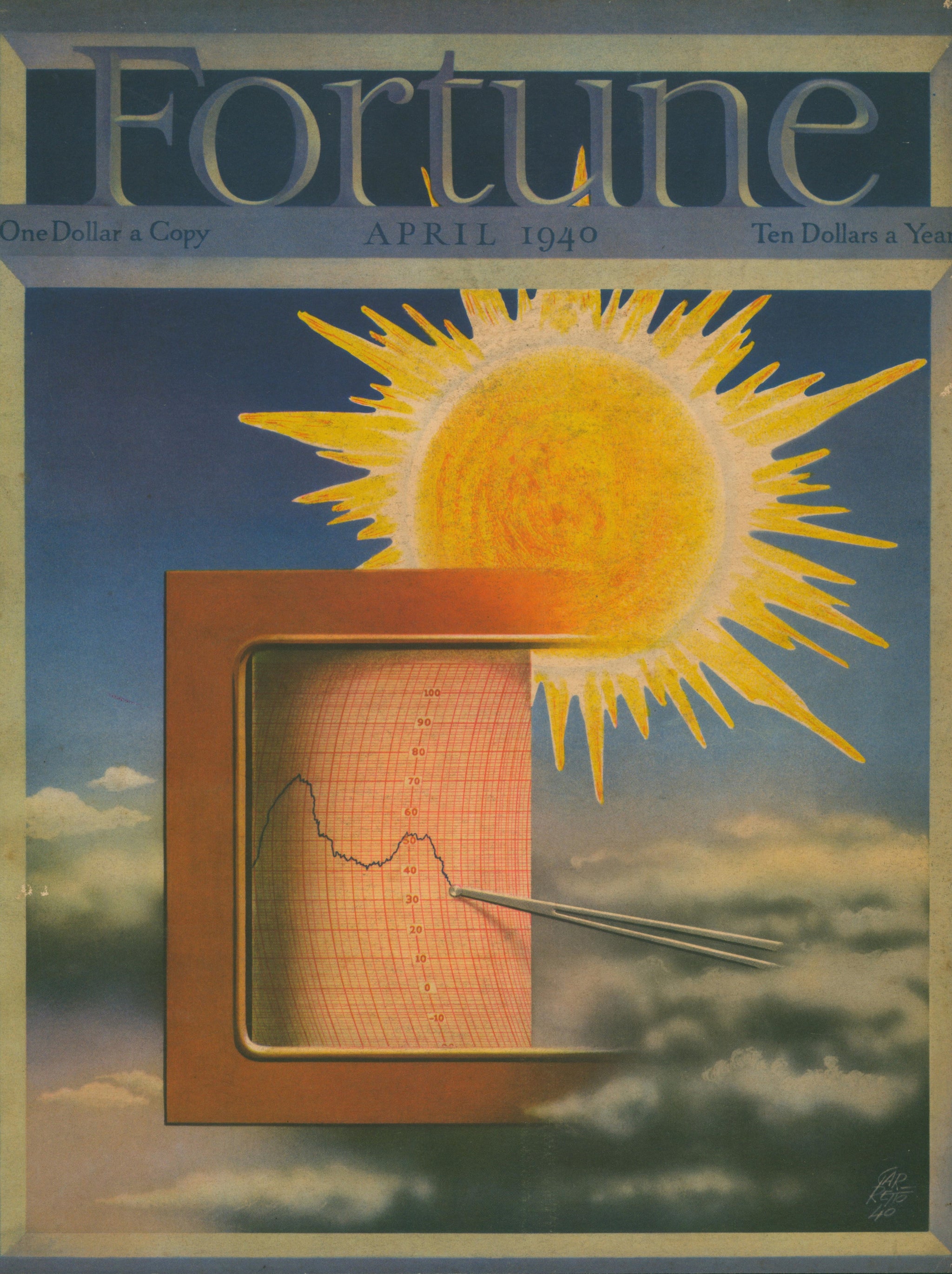The magazine cover features the title "Fortune" at the top in gray, 3D lettering with a small, blue text underneath indicating the price as "One dollar a copy." The center of the title area reads "April 1940," and the right side states "Ten dollars a year." The cover itself is encased in a tannish-gray border. Dominating the visual is an illustration of a radiant sun design with yellow and orange swirls, encircled by a white ring and surrounded by jagged, bright yellow beams. Below the sun, a telegraph machine, depicted only partially with a C-shaped wooden frame, draws a jagged blue line across a red grid, symbolizing a seismograph’s recording. This device gradually fades away towards the right, with grayish blue clouds and sky forming the backdrop. The bottom right corner features an unreadable signature, adding an artistic touch.